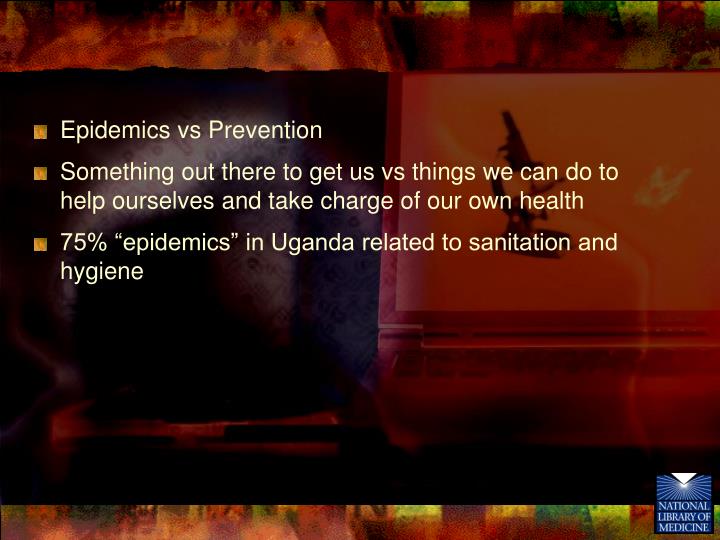The image displays an educational slide with a textured background featuring abstract reddish-orange and green patterns, possibly representing the colors of Africa. The slide contains three bullet points in white text: "Epidemics vs. Prevention," "Something Out There to Get Us vs. Things We Can Do to Help Ourselves and Take Charge of Our Own Health," and "75% Epidemics in Uganda Related to Sanitation and Hygiene." In the lower right corner, the blue and white logo of the National Library of Medicine is prominently featured.